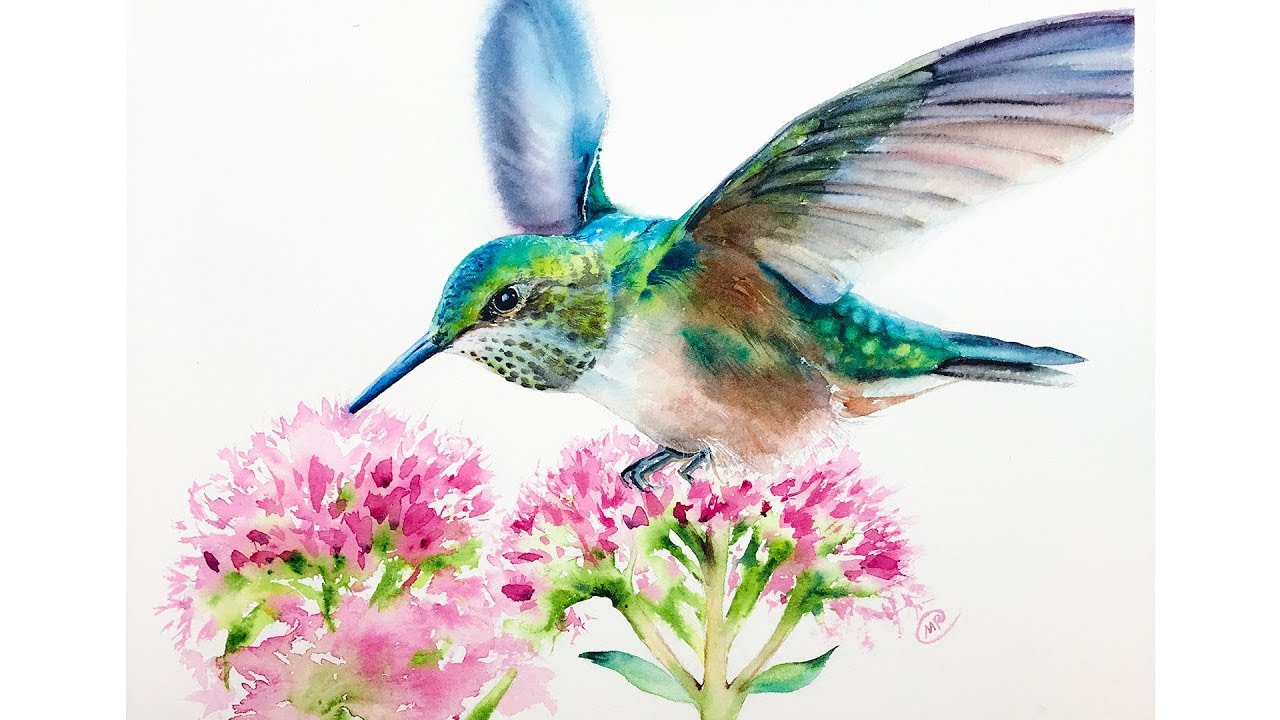This is a detailed watercolor painting of a lifelike hummingbird interacting with a cluster of pink flowers. The scene is set against a white background, with the hummingbird positioned in flight, its beak partially obscured as it dips into one of the small pink blossoms located in the bottom left quadrant of the image. The pink flowers have green stems and resemble clover blossoms with their tiny, delicate petals. The hummingbird itself is beautifully detailed, with a green head adorned with a blue crown, blue wings extended outwards, and a mix of green and blue on its back. Its belly showcases a blend of white and brown hues. Notably, there is some red shading under its wings, a distinctive green stripe above its eye, and black eyes, while its blue beak is subtly spotted under the chin. The bird hovers gracefully just above another similar bloom, capturing a moment of natural elegance in vibrant colors.